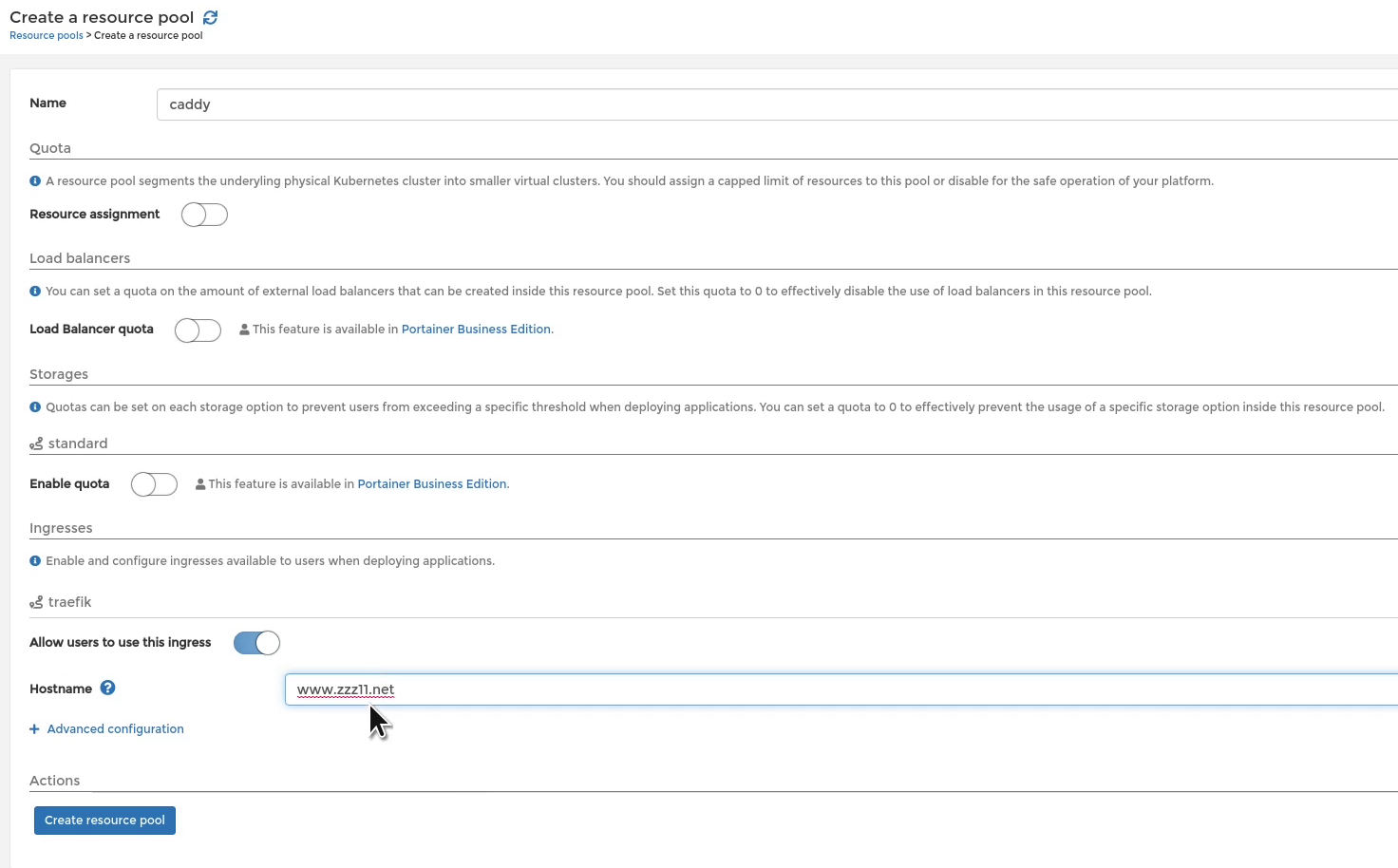**Detailed Caption:**

The screenshot depicts a detailed interface for creating a resource pool within a Kubernetes management platform. At the top, the page title "Create a Resource Pool" is displayed, accompanied by an icon featuring a circular arrow pattern reminiscent of the Ouroboros symbol. Directly below, the heading "Resource Pools" is present, followed by a caret symbol that expands the submenu labeled "Create Resource Pool."

A gray line divides this section from the questionnaire-style form below. The first input field, bolded and labeled "Name," has the name "Caddy" (spelled C-A-D-D-Y) already entered. Below this is the "Quota" section, accompanied by an information icon providing descriptive text about resource pools. It notes that resource pools segment the physical Kubernetes cluster into smaller virtual clusters and recommends assigning a capped limit of resources for safe platform operations.

The "Resource Assignment" section follows, marked by a bold heading. Here, a slider button, currently positioned to the left, allows adjustment of resource limits. The next section addresses "Load Balancers," once more featuring an information icon that explains the ability to set a quota on external load balancers within the resource pool. It mentions that a zero quota effectively disables load balancers. This segment includes another slider positioned to the left, with a disclaimer indicating the feature is exclusive to the Portainer Business Edition.

Further down, the "Storages" section is outlined with an information icon. This area allows setting quotas on various storage options to prevent users from surpassing specific thresholds when deploying applications. The "Standard" storage option is listed first, with a bolded "Enable Quota" heading and another left-slid button, again noting the feature’s availability in Portainer Business Edition.

Next, the "Ingresses" section is presented. An information icon details that enabling and configuring ingresses makes them available to users for application deployment. A unique symbol resembling a coiled snake (possibly for the ingress controller Traefik, spelled T-R-A-F-I-K) introduces the sub-section. It includes a bold "Allow Users to Use this Ingress" with a right-slid button indicating it is enabled. Beneath, the "Host Name" field, featuring a blue question mark for additional information, contains the user-entered URL www.zzz11.net. An adjacent plus sign and the "Advanced Configuration" link suggest further customizations.

Finally, the "Actions" section at the bottom houses a turquoise blue button labeled "Create Resource Pool," ready for the user to submit their configurations.